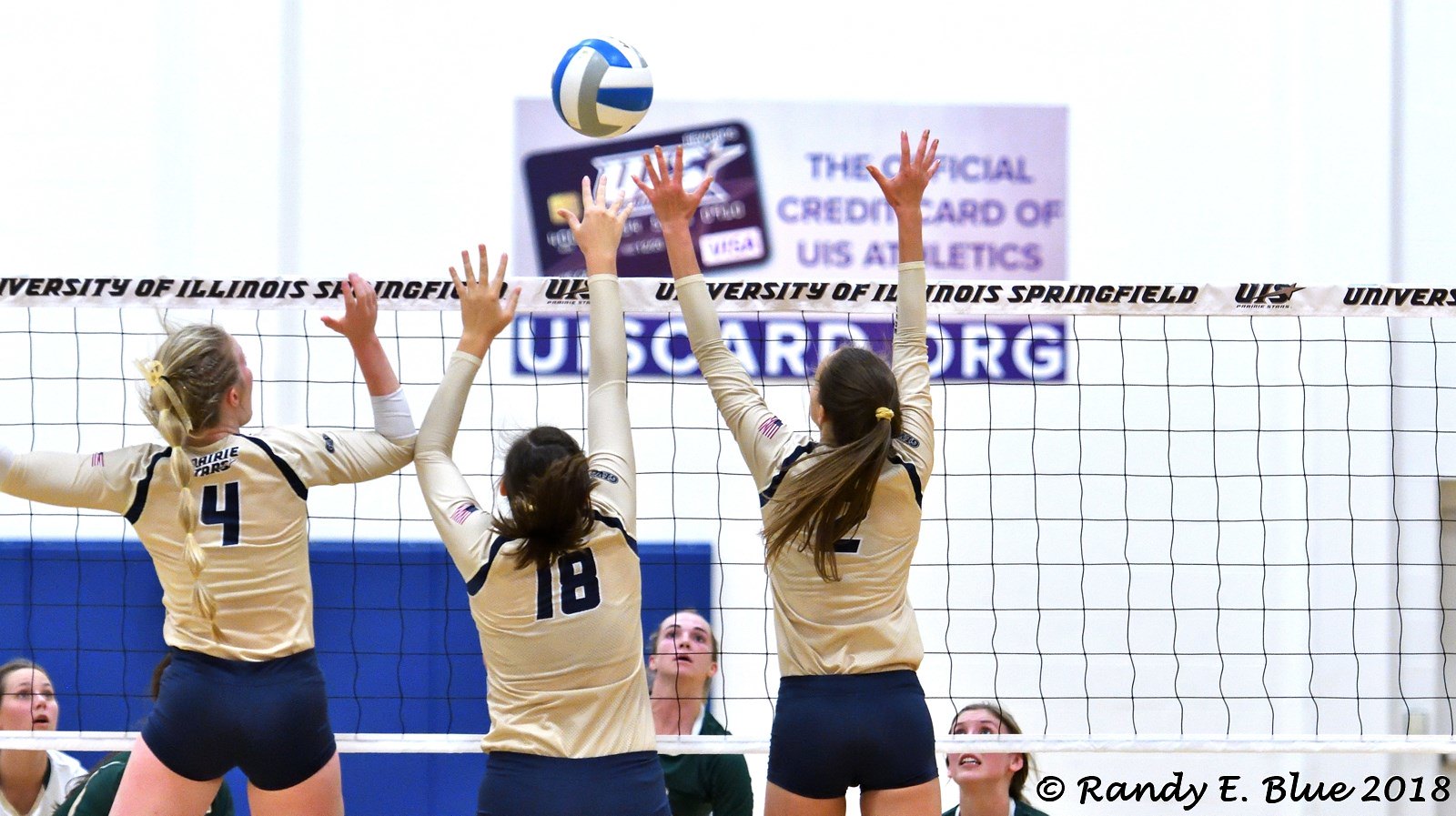In this dynamic image of a women's volleyball game at the University of Illinois Springfield, three girls from the team are captured mid-jump, intensely reaching for a white, blue, and green striped volleyball soaring above the net. Each girl wears a cream-colored long-sleeved jersey and dark navy shorts. From left to right, their jerseys are numbered 4, 18, and 2. The white net, prominently marked with "University of Illinois Springfield," separates them from three opposing team members in dark green shirts who are crouched and focused on the ball. In the upper center of the photo, an advertisement for the official credit card of UIS Athletics, uscard.org, is visible, featuring a drawing of the card and a blue border around the text. The background, though blurry, consists of a white wall with some visible blue elements. At the bottom of the image, a copyright reads "Randy E. Blue, 9th, 2018," documenting the moment of action and concentration during the heated match.